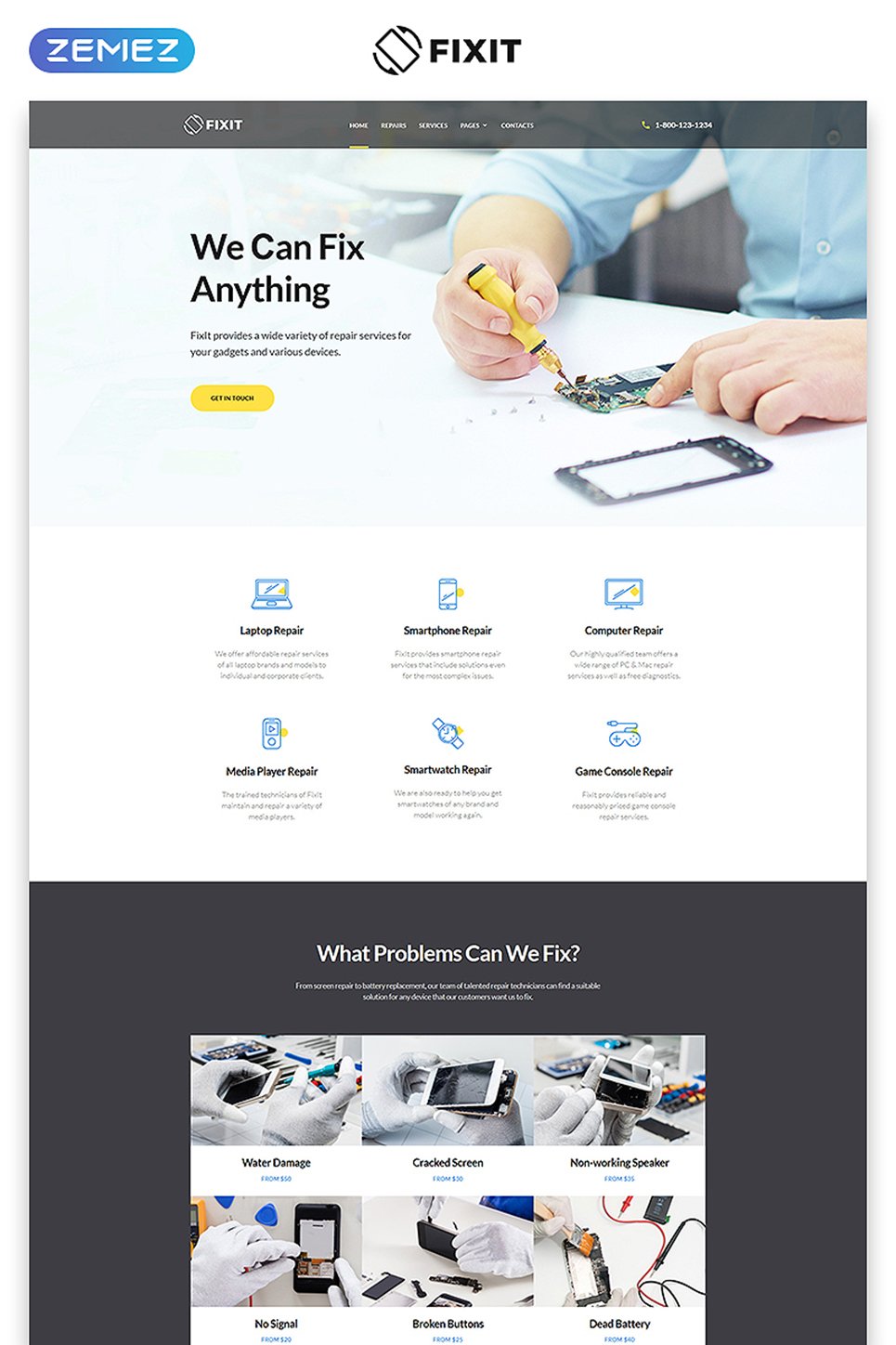In this image, we see a detailed screenshot of a website. The upper left corner features the website name "Zemes" in blue text against a white background. To the right, in bold black text, is the phrase "Fix It." Beneath this, there is a dark gray banner displaying "Fix It" alongside a cell phone icon. The banner includes a menu that reads from left to right: Home, Repairs, Services, Pages (with a dropdown menu), and Contacts. In the upper right corner of the banner, there is a phone number: 1-800-123-1234.

Below the banner, there is a color photograph depicting a white table with a dismantled cell phone on it. Two hands are seen working on the cell phone, and the person behind the desk is wearing a blue button-down, long-sleeved shirt. To the left of the photograph, in large bold black text, are the words "We Can Fix Anything." Beneath this header, there are various repair services listed: "Laptop Repair, Smartphone Repair, Computer Repair." Further down, in smaller black text, additional services are mentioned: "Media Player Repair, Smartwatch Repair, and Game Console Repair."